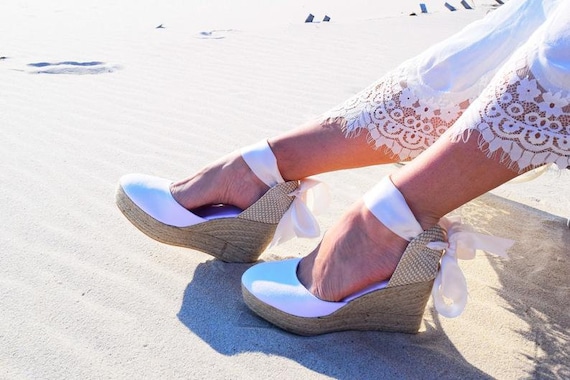This is a close-up, detailed photography image of a woman's feet adorned with brand new wedge platform sandals, perfect for an advertisement. The sandals feature a brown, wickered platform base and a pristine white canvas top, complemented by a white ribbon that forms large, prominent bows to secure around the ankles. Her feet are elegantly pointed downward, suggesting a relaxed, sitting position on light brown sand, evidenced by the clearly visible shadows cast on the ground. Nestled in a beach setting, the model is also wearing a white dress, adding a touch of grace to the overall composition.